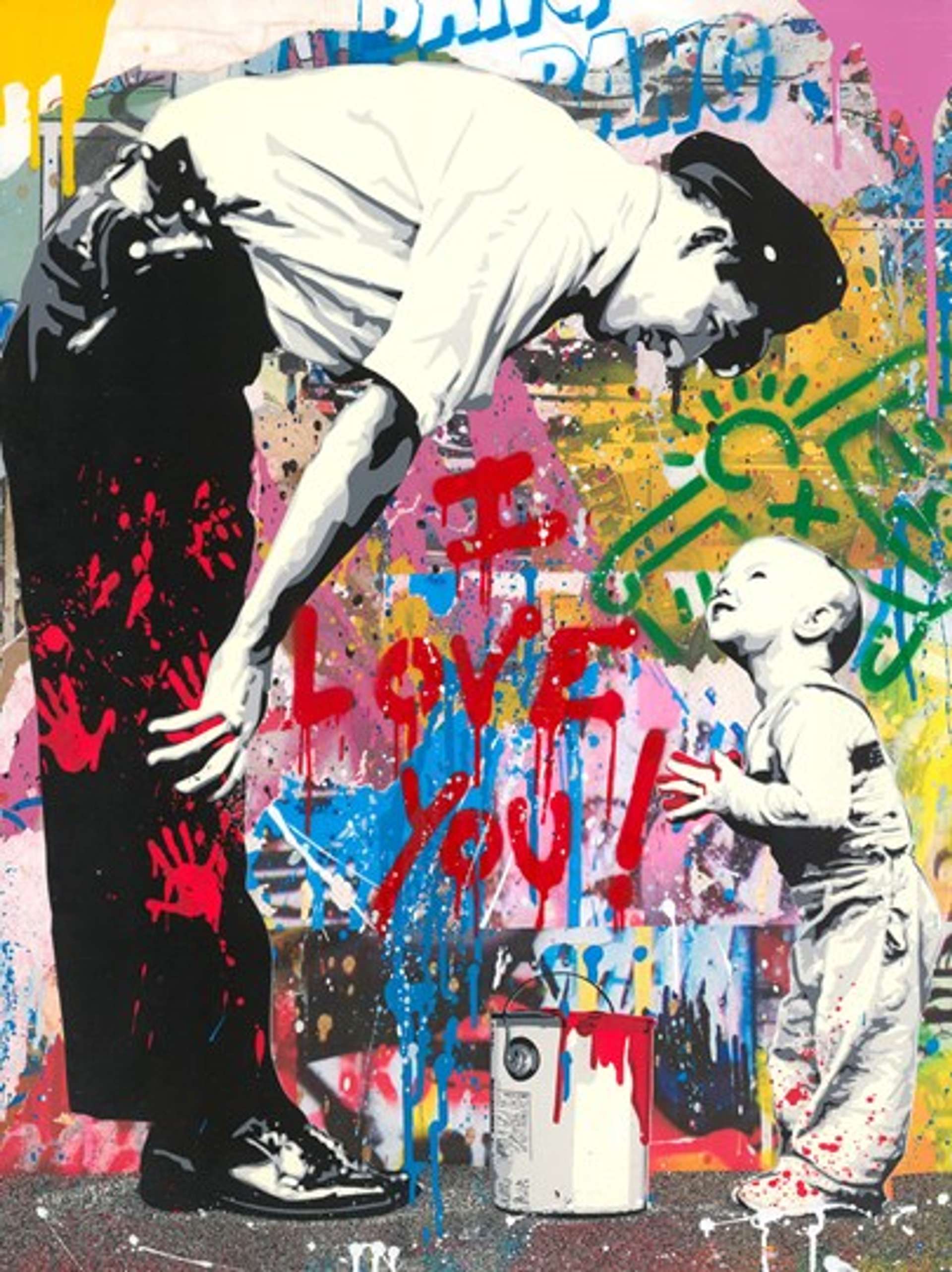The image portrays a poignant and vibrant scene that blurs the lines between photography and painting, featuring a vertically rectangular composition without a definitive border or background. Central to the artwork is a police officer, distinguished by his shiny black shoes, black pants, white short-sleeved shirt, and police cap. He stands with a gun holstered at his side, bending slightly to engage with a small boy who looks up at him. The boy and the officer are positioned around a can of red paint placed on the ground between them, with both figures intricately detailed. Notably, red handprints are smeared over the officer’s pants, and traces of red paint are visible on the boy’s clothing. Above them, the words "I love you!" are vividly painted in red, standing out against a chaotic backdrop of multicolored graffiti that embellishes the wall behind them. This richly detailed image captures a compelling moment of interaction, infused with a raw, emotional undertone and an artistic blend of styles and elements.